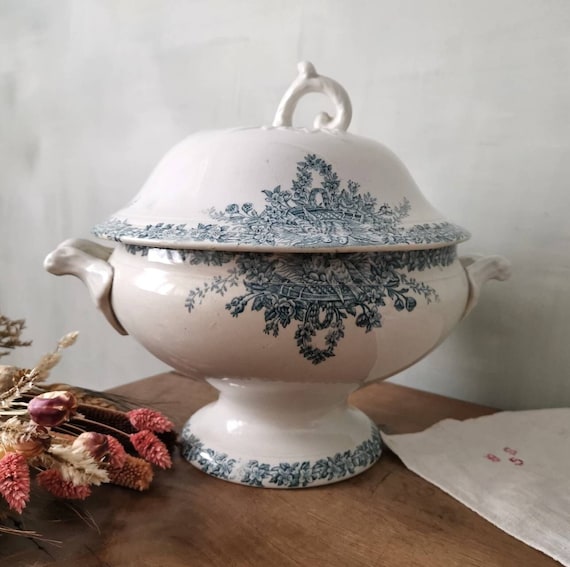This photograph features an ornate porcelain container, resembling an old-fashioned English-style teapot with a lid. The teapot, set on a brown wooden table, displays intricate blue floral engravings that embellish its white surface. It has handles on either side, and the lid, adorned with a handle that curves like a vine or twig, sits gracefully on top. Surrounding the teapot are a few key elements: to the left, a cluster of dried flowers in shades of pink, ivory, and a hint of purple; and to the right, a white napkin embroidered with letters. The setting is completed by a blank white wall in the background, offering a striking contrast to the antique aesthetic of the scene.